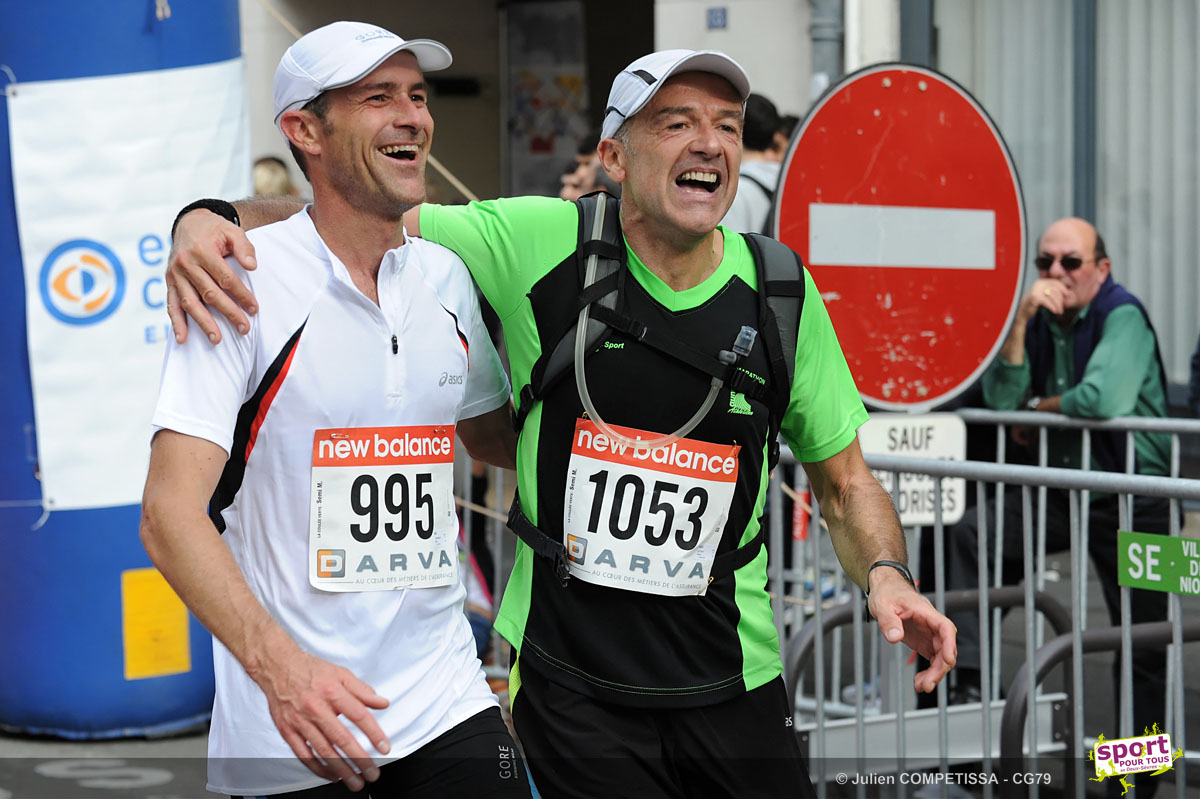In the foreground of this photo, two men, who appear to be marathon or triathlon participants, are smiling and embracing each other in a celebratory manner, as if they have just finished a race. The man on the left, wearing a white athletic shirt and a white bicyclist cap, has a race bib with the number 995 and the word "New Balance" printed across the front. He appears to be in his 30s. The man on the right, who looks to be in his 60s, is dressed in a black and lime green shirt with a white cap, and his race number is 1053, also featuring "New Balance." His shirt includes a hydration pack, suggesting endurance sports involvement.

The man on the right has his arm draped around the shoulders of the man in white, while the man in white's left arm encircles the waist of his companion. Both men are beaming with joy.

Behind them, a distinctive red "Do Not Enter" sign with a white dash stands out, indicative of European signage, potentially placing the scene in France, as inferred from other signage in the background. Gray crowd-control fencing supports a few spectators, including a bald man with sunglasses leaning casually against it. He wears a black vest over a green shirt and watches the two athletes with an appreciative expression. Additional details in the background include a partially visible blue inflatable column and various banners adding to the event's atmosphere. The copyright credit, indicating "© Julien COMPETISSA. CG 79," and the logo "SPORT" in maroon on a white background, appears at the bottom right corner of the image.